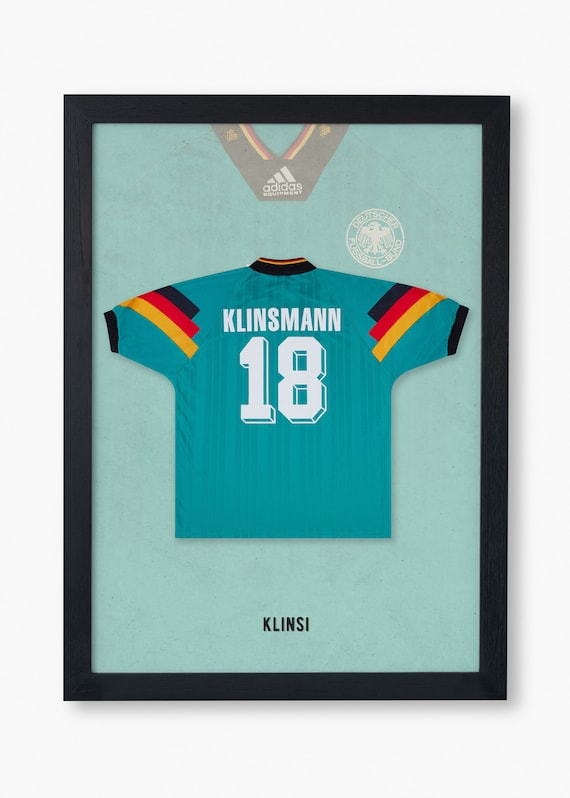This is a detailed photograph of a framed teal jersey with notable elements and decorations related to Germany. The jersey prominently displays the name "Klinsmann" in bright white letters across the chest, accompanied by the number "18" below it. The number "18" features a dark blue shadow creating a 3D effect. The shoulders of the jersey are adorned with three diagonal stripes representing the German flag: a short black stripe, followed by a mid-length red stripe, and ending with a longer yellow (or orange) stripe. The V-neck of the jersey is accented with a black trim, separated by a white stripe, and then topped with another black stripe.

The frame itself is simple and black, providing a stark contrast to the light teal background within it. Additionally, inside the frame near the top, there's a black ribbon bearing the iconic Adidas logo, designed to resemble a mountain with three stripes. The Adidas branding also features smaller, black, red, and yellow stripes, echoing the German flag colors. Below the jersey, still within the frame, the name "Klinsi" is written in black text against the teal backdrop. 

A small seal sits on the top right of the inner frame, although its details are difficult to discern. The entire assembly is mounted on a plain white wall, ensuring all focus is on the framed jersey.